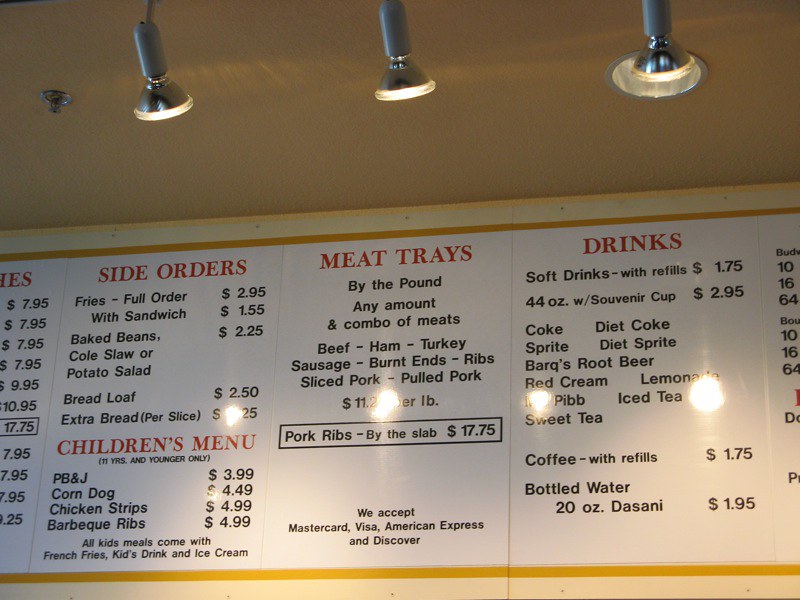The image features a rectangular, white menu mounted on a wall, accentuated with a fine yellow border followed by a cream border. A very light yellow border serves as the final edge at the top. Above the menu, the ceiling is painted in a cream color. The menu itself is detailed with various items available for purchase, with prices listed in dollars. 

"Side Orders" is prominently displayed in red lettering on the white background, listing items such as fries, baked beans, coleslaw, bread loaf, and extra bread. Below this, the "Children's Menu" is also highlighted in red, featuring options like corn dog, chicken strips, barbecue ribs, and PB&J. Further sections include "Meat Trays" and "Drinks," each denoted in red text.

Illuminating the menu are three spotlights suspended from the ceiling, casting reflections on its surface. Additionally, a recessed light is situated next to the third spotlight, providing further illumination. Intriguingly, there is only one recessed light amidst the three spotlights, a detail that stands out.

In the top left corner of the image, the ceiling houses a sprinkler system designed to activate in case of a fire. This sprinkler is built into the roof, providing a functional safety feature in the setting.